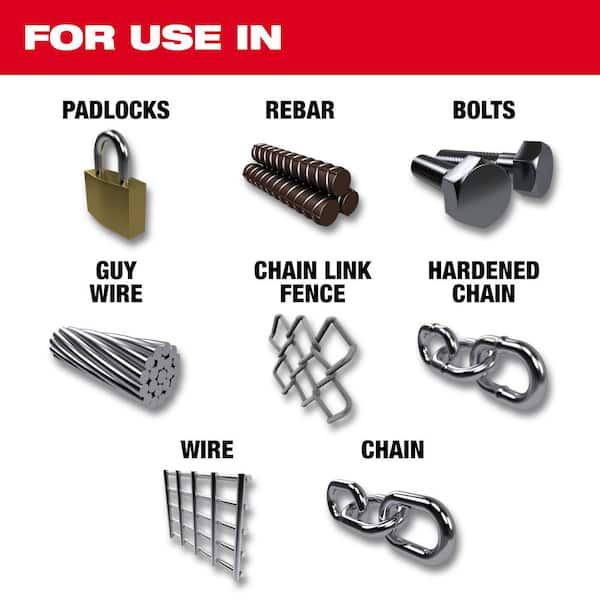This digital poster features a collection of metallic objects displayed on a white background, with descriptive text and images organized neatly. At the top, a bold red horizontal strip runs across the image, with the phrase "For Use In" prominently displayed in thick, white block letters on the left-hand side. Below this strip, there are three rows of items. The top two rows each contain three items, while the bottom row has two.

Each item is accompanied by its name written in smaller black block letters above its corresponding image. The depicted items, from left to right and top to bottom, are:

1. **Padlocks** – A silver padlock with a gold bottom.
2. **Rebar** – Three brown bars with silver accents.
3. **Bolts** – Silver bolts.
4. **Guy Wire** – A depiction of a silver guy wire.
5. **Chain Link Fence** – A section of grey chain link fence.
6. **Hardened Chain** – Three links of a hardened chain.
7. **Wire** – Silver wire.
8. **Chain** – Three links of a chain.

The images for "Hardened Chain" and "Chain" appear nearly identical, emphasizing the metallic nature of the objects showcased in this informative guide.